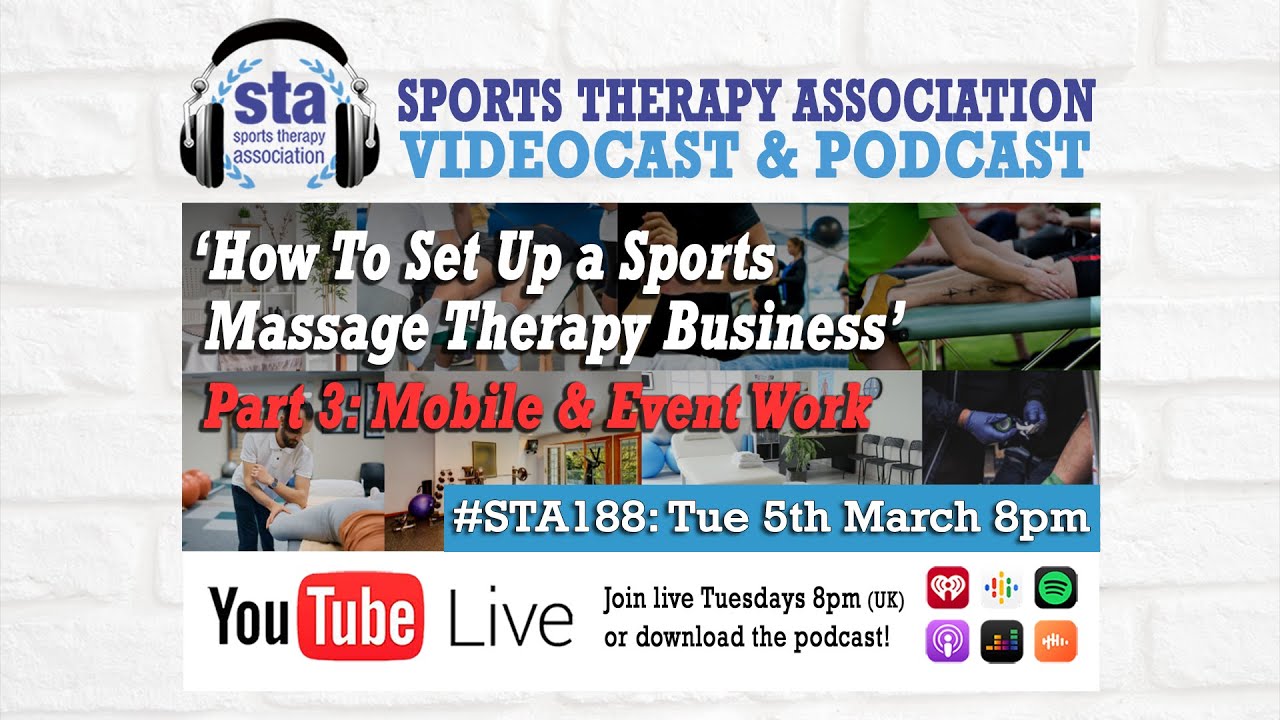This rectangular advertisement, oriented horizontally, promotes a YouTube Live event hosted by the Sports Therapy Association. The backdrop features a white-painted brick wall, giving it a clean and modern aesthetic.

At the top of the advertisement, the words "STA Sports Therapy Association" appear prominently with a surrounding graphic of headphones, emphasizing the audio-visual nature of the event.

Below this, the text "Sports Therapy Association" is rendered in a darker blue, followed by "Videocast and Podcast" in a lighter blue, highlighting the multimedia format of their content.

Central to the ad is a specific promotional box featuring the title "How to Set Up a Sports Massage Therapy Business" in white text. This is accompanied by a subtitle in red text, "Part 3: Mobile and Event Work," indicating that this is the third installment of an ongoing series.

Further down, a blue box with white text provides detailed scheduling information: "#STA188, Tuesday, 5th March, 8 p.m."

At the very bottom of the advertisement, another white box with dark text reads "YouTube Live" with the iconic red and white 'tube' logo. It invites viewers to "Join Live Tuesdays, 8 p.m. UK" or download the podcast for later listening.